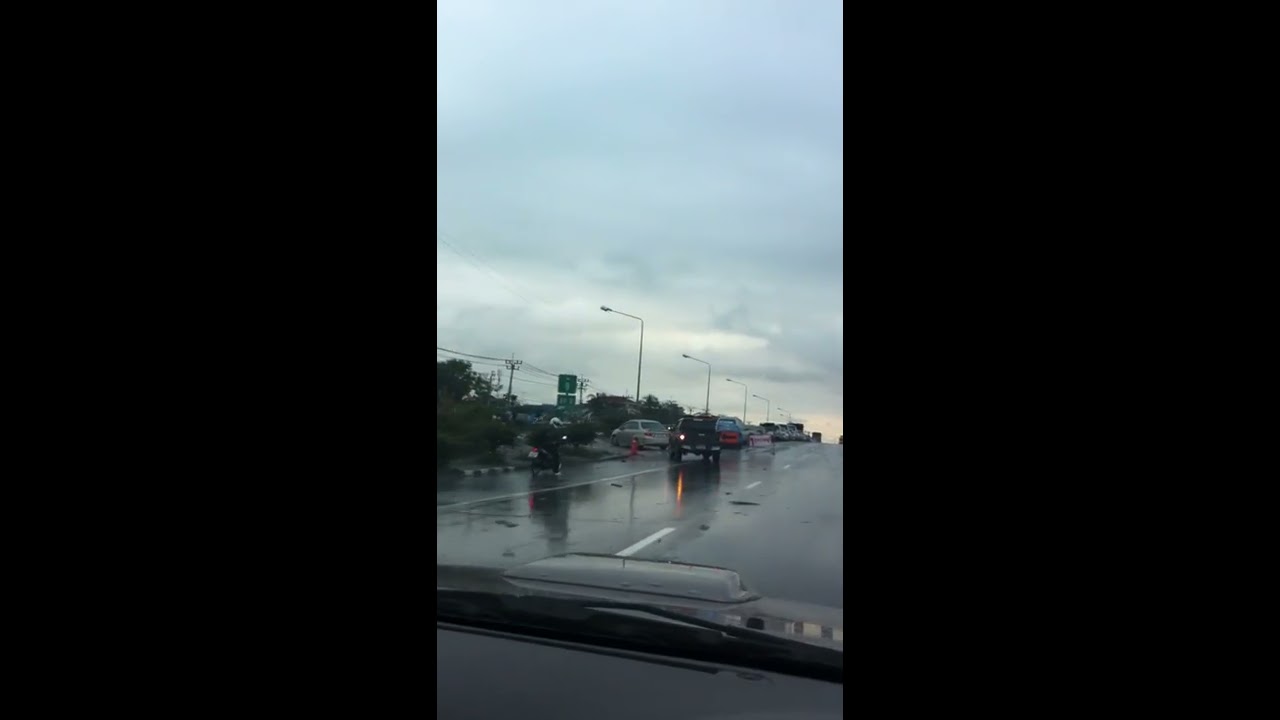The image depicts a rainy, overcast outdoor scene captured from inside a moving car during early morning or dusk. The car, with its shiny dashboard at the bottom edge of the frame, is driving along a wet, multi-lane road. In the foreground, the road features a white dotted center line and wet pavement, suggesting recent rain. The scene is framed on the left and right by vertical black borders, creating a central focus.

In the background, several vehicles, including a truck and a white car, are seen traveling away from the viewer. To the left, a small, ambiguous parking lot or turning road is visible, along with distant trees. The sky is filled with thick, gray clouds, adding to the dim, overcast ambiance. Streetlights line the road, and indistinct business signs can be spotted, though their text is unreadable.

Further details include an orange light glowing faintly in the far background and various colors visible throughout the scene, such as shades of blue, white, gray, green, black, tan, red, and purple. On the shoulder of the road, a man wearing a white helmet and black suit rides a motor scooter, passing a fire hydrant. Near him, two vehicles—a silver sedan and a black pickup truck with a broken right taillight—are attempting to make a left turn. A red arrow sign points left, accompanied by an unreadable pink sign. Beyond this, a row of parked vehicles and street lamps continues into the distance, all under the cloudy sky.